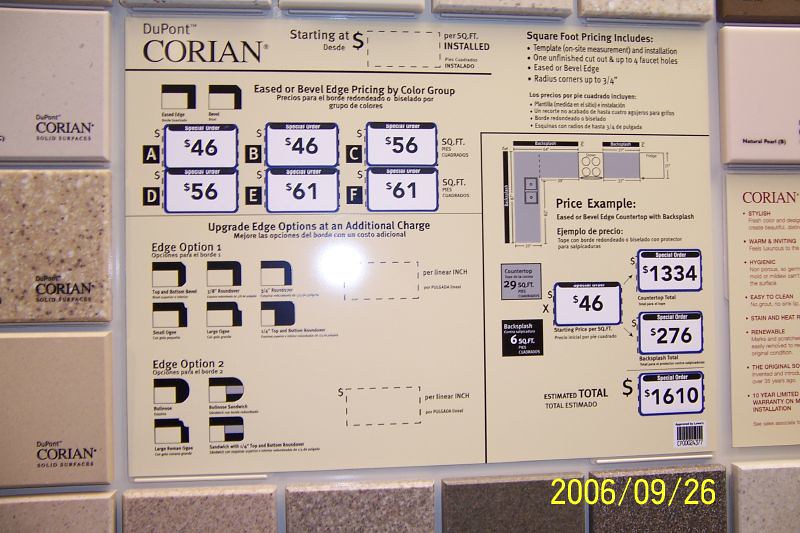The image displays a document with a primary date indicated as "2006/09/26" in the top right corner. The top left corner of the document features the brand name "DuPont," surrounded by several instances of the word "Korean" positioned at the top left, left, bottom left, and right sides. There is also a marked area indicating prices structured in a square format, listing amounts such as $46, $46, $46, $46, $61, $61, and a series of repetitive prices like $6, $6, $6, $1, $6, $1. Towards the bottom of the document, a note specifies "Upgrade edge options with an additional charge," labeled specifically as "Edge Option 2." On the far right, it mentions a "Price Example" followed by incremental listings such as $1, $2, $4, and multiple instances of $4 leading to an "Estimate Total."